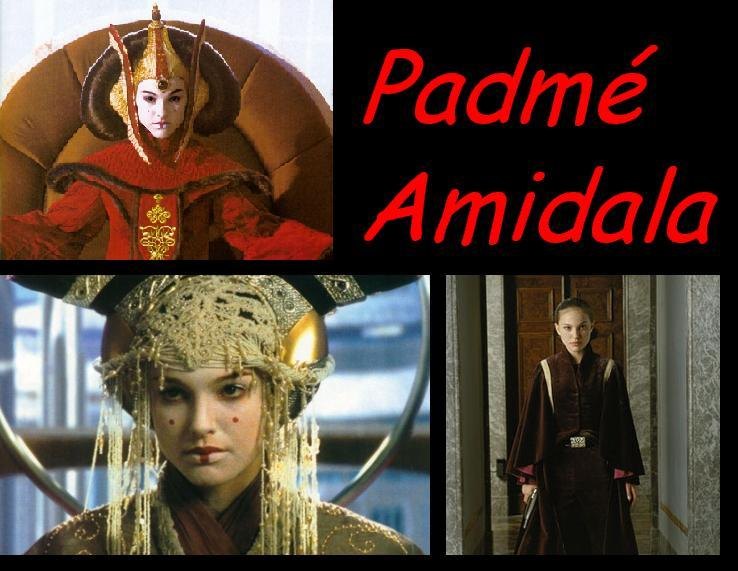The image features Padmé Amidala, a character from Star Wars portrayed by Natalie Portman. It includes three distinct portrayals of her from different scenes. 

In the upper left, Padmé is depicted from the earlier movies like *The Phantom Menace*. She is seated on what appears to be a brown chair or throne, adorned in a red robe-like gown. Her hair is styled in brown loops, and her face is painted white with red accents, including red dots and lipstick, and she wears a large golden crown.

Below this, the middle image shows her similarly attired with white face paint and red facial markings, including the red dots and lipstick. Her expression is a blank stare, emphasizing the makeup and grandiose headpiece she is donning.

The bottom right image presents a contrasting depiction. Here, Padmé wears a brown or purple robe with white stripes and has brown hair without any intricate styling or makeup. She holds a gun or blaster in her right hand and stands in front of a doorway, suggesting a more action-oriented scene from the movies.

The top right corner of the image has text identifying her as "Padmé Amidala."